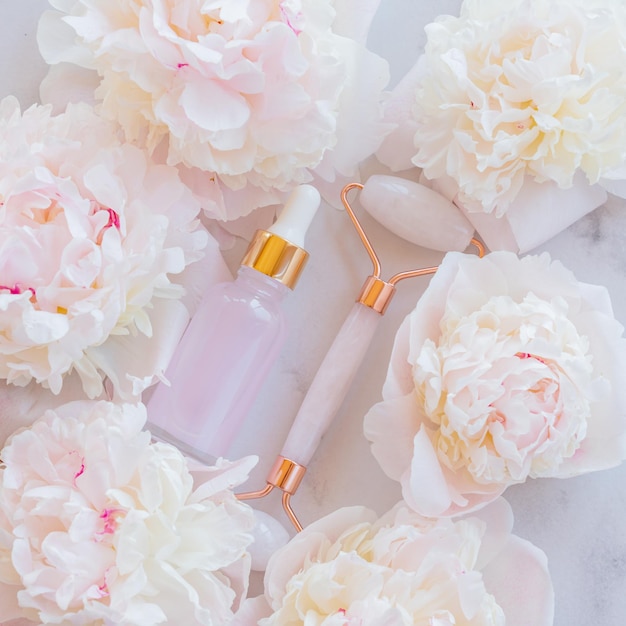In this brightly lit photograph set on a white marble table, six pale white to slightly pinkish roses are arranged in a circle along the outer edges. At the center, two cosmetic products are prominently displayed on a white background that closely matches the hues of the surrounding flowers. The left item is a bottle with a white applicator tip, topped with a golden metal band, suggesting it contains a serum or beauty liquid. On the right is a face roller, designed for skin massage, featuring a white marble handle with gold accents, a metal connector, and a white bead that allows it to roll. The overall aesthetic of the photograph emphasizes purity and elegance, highlighting the self-care tools amidst the soft floral arrangement.